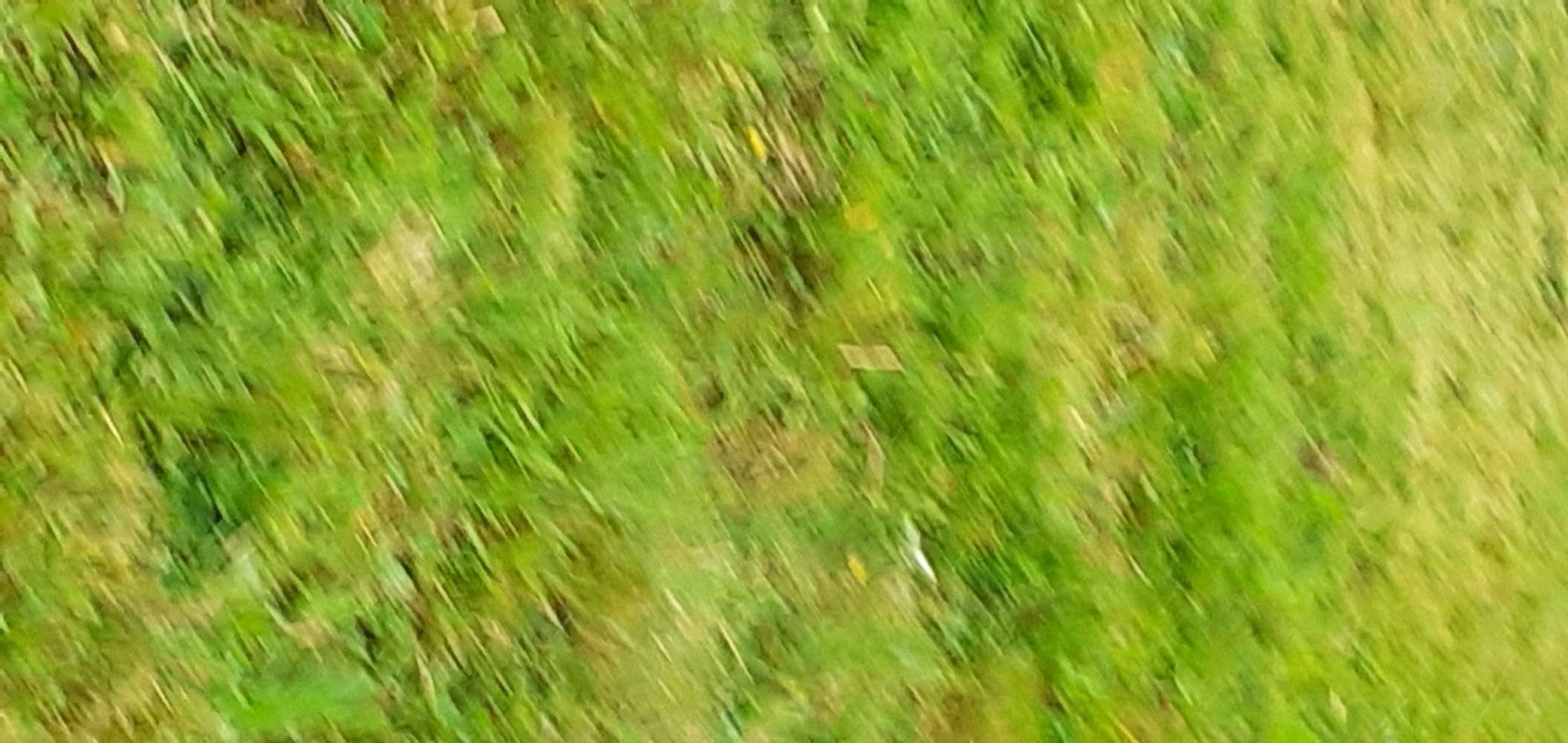A close-up, slightly blurred photograph of a mixed grass lawn in early spring. The image captures a variety of grass types in different stages of growth: bright green blades mingling with yellowing strands, and scattered dark patches hinting at underlying soil. The grass appears to have been mowed within the last two weeks, yet new growth suggests it may require another trim soon. Amidst the mix, individual blades of both green and yellow grass stand out, adding to the natural, unmanicured appearance of the lawn.